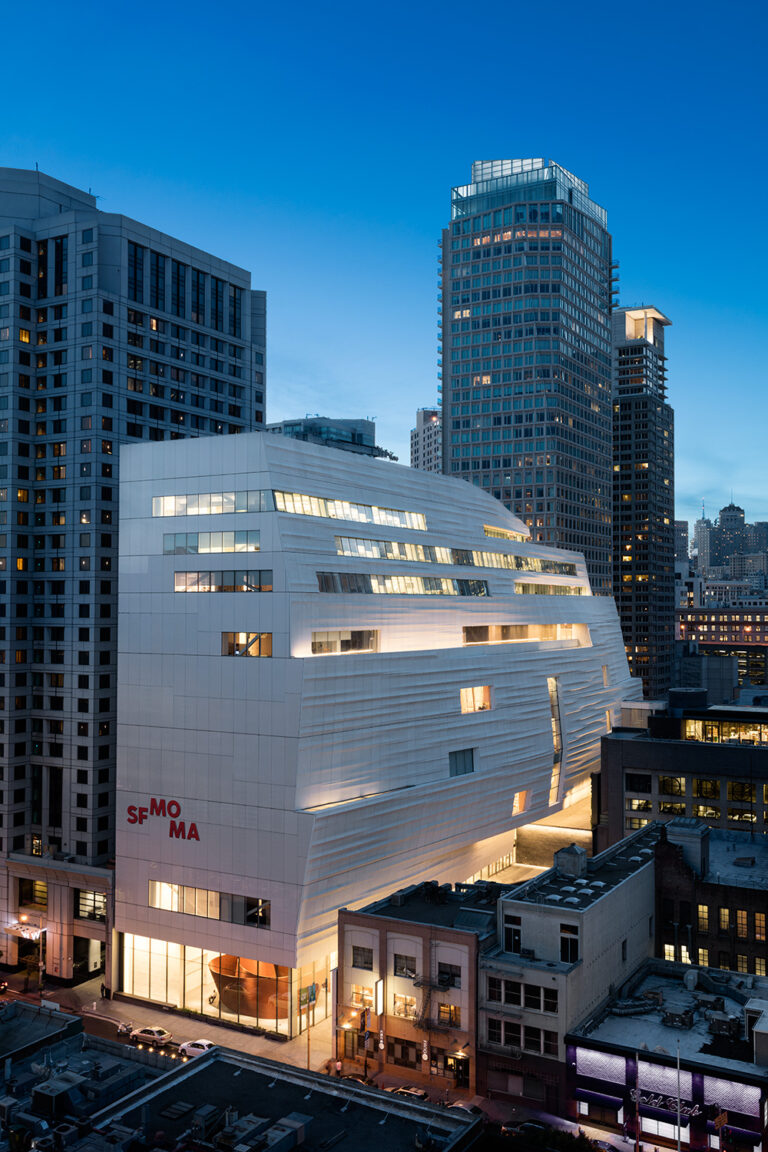The image showcases the San Francisco Museum of Modern Art (SF MoMA) prominently in the center, captured during late dusk or twilight with a deep blue sky hinting at the sun below the horizon. The main building is an artistically shaped, multi-level white structure with "SF MoMA" displayed in red letters on its facade. The well-lit first floor reveals a lobby with an artistic installation that appears round and brown, reminiscent of a hat. Surrounding the museum are taller gray and lavender-hued skyscrapers, hinting at a bustling downtown San Francisco. Streets are adorned with a variety of vehicles, including white and light yellow cars, and illuminated city lights bring the scene to life. The bottom left corner of the image features what appears to be an apartment building, adding a residential touch to the urban landscape.